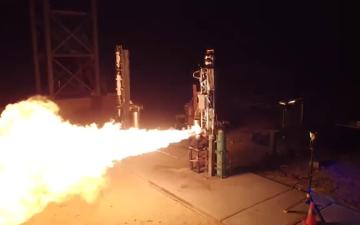The image shows a tall, possibly metal structure centrally positioned on a concrete floor. Next to it, there is a large green tank. The structure is emitting a dramatic jet of flame from its lower third, projecting to the left side of the image, which is the main focus. This scene, captured in a somewhat unclear photograph taken at night, creates a surreal and intense visual, with the edges cloaked in darkness. To the right of this structure, a small light post is visible, while a similar trellis-like structure stands off to the left. The fiery jet and the ambiguous details suggest a possible rocket launch or a gas explosion, although the image's quality makes finer details difficult to discern.